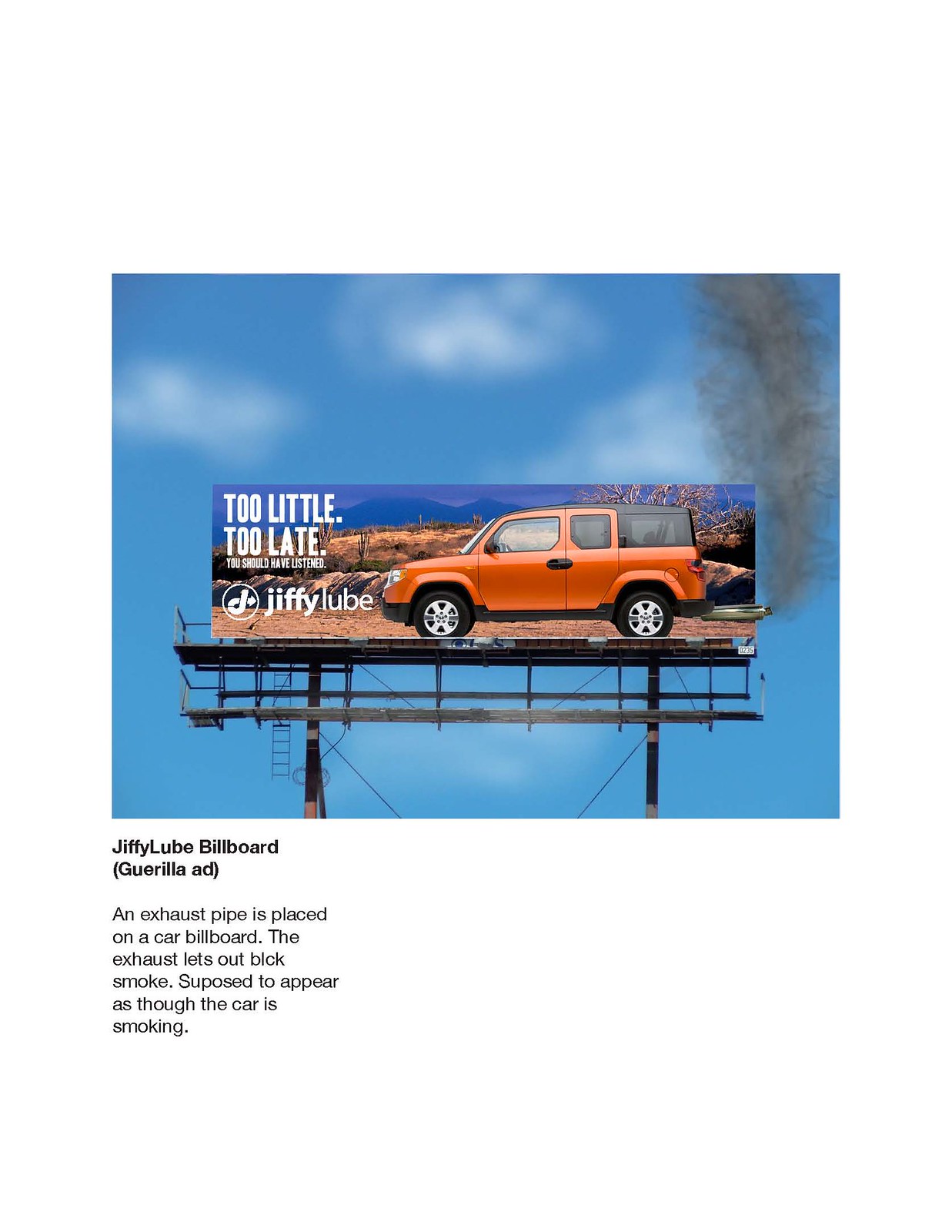The image portrays a Jiffy Lube billboard set in a desert landscape with a vast blue sky backdrop and three puffy white clouds. The billboard features an orange, boxy vehicle with silver rims driving to the left, which might have a camper attached to its bed. The text "Too Little, Too Late. You Should Have Listened." is prominently displayed alongside the Jiffy Lube logo. A key feature of the billboard is a real exhaust pipe extending from the rear of the vehicle depicted in the ad, spewing black smoke into the sky to create the visual illusion that the car is emitting exhaust. The ground below shows brown terrain with sparse vegetation, including cacti. In the bottom left corner, text reads: "Jiffy Lube Billboard, Gorilla Ad. An exhaust pipe is placed on a car billboard. The exhaust lets out black smoke supposed to appear as though the car is smoking." This clever design integrates elements of concept art and real-world components to drive home its message.